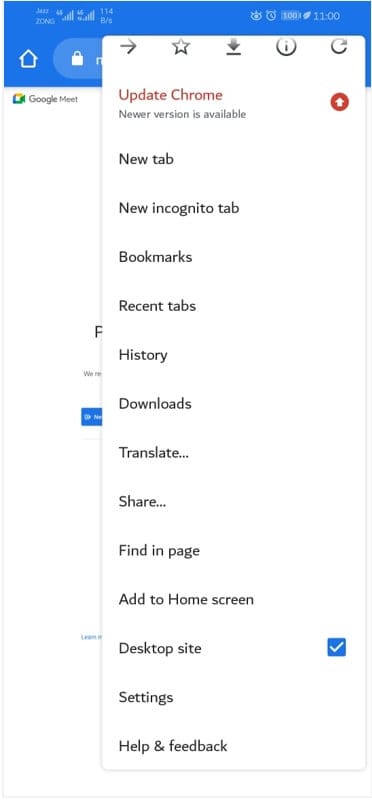A smartphone screen displays the Google Meet app. A pop-up window prompts the user to update Chrome, indicating that a newer version is available. The pop-up also provides a variety of options including New Tab, New Incognito Tab, Bookmarks, Recent Tabs, History, Downloads, Translate, Share, Find in Page, Add to Home Screen, Desktop Site, Settings, Help, and Feedback. The phone's status bar is visible at the top of the screen, showing icons such as an alarm clock and the current time, which is 11:00.